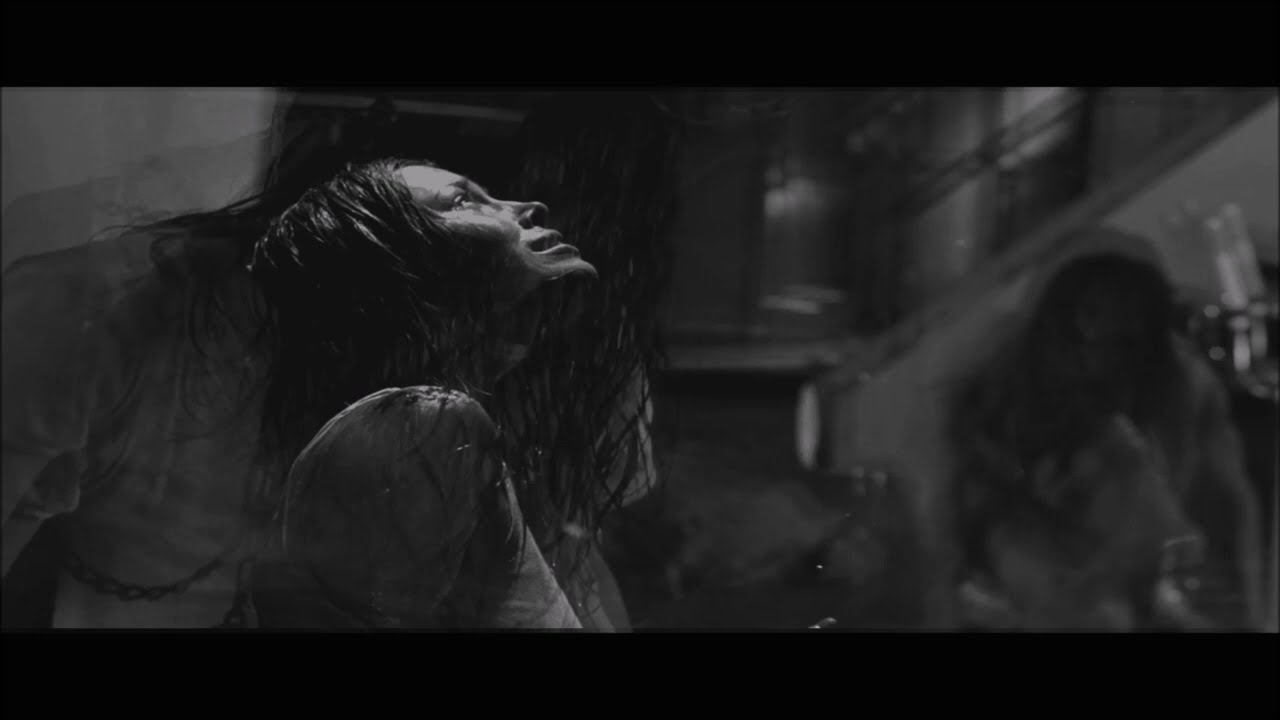In this striking black and white photograph, a young woman with dark, wet hair stands in what appears to be a gloomy, rain-soaked environment. Her head is tilted back as she looks upwards, her expression conveying distress and possibly pain, with tears streaming down her face. She is clad in a white tank top, and only her shoulders and above are visible. Illuminated by a nearby streetlight or possibly another strong light source, the rain glistens on her skin, casting light on her forehead and right cheek. The background is shrouded in shadow and blur, adding an eerie atmosphere, with vague outlines suggesting a mix of outdoors and urban environment, perhaps near an old apartment building. Subtle, transposed images create a surreal, overlapping effect, with hints of additional figures and objects like a chain, a window, and a dim sconce. The scene possesses an artistic, almost cinematic quality, intensified by the presence of ominous shapes and dark tones.